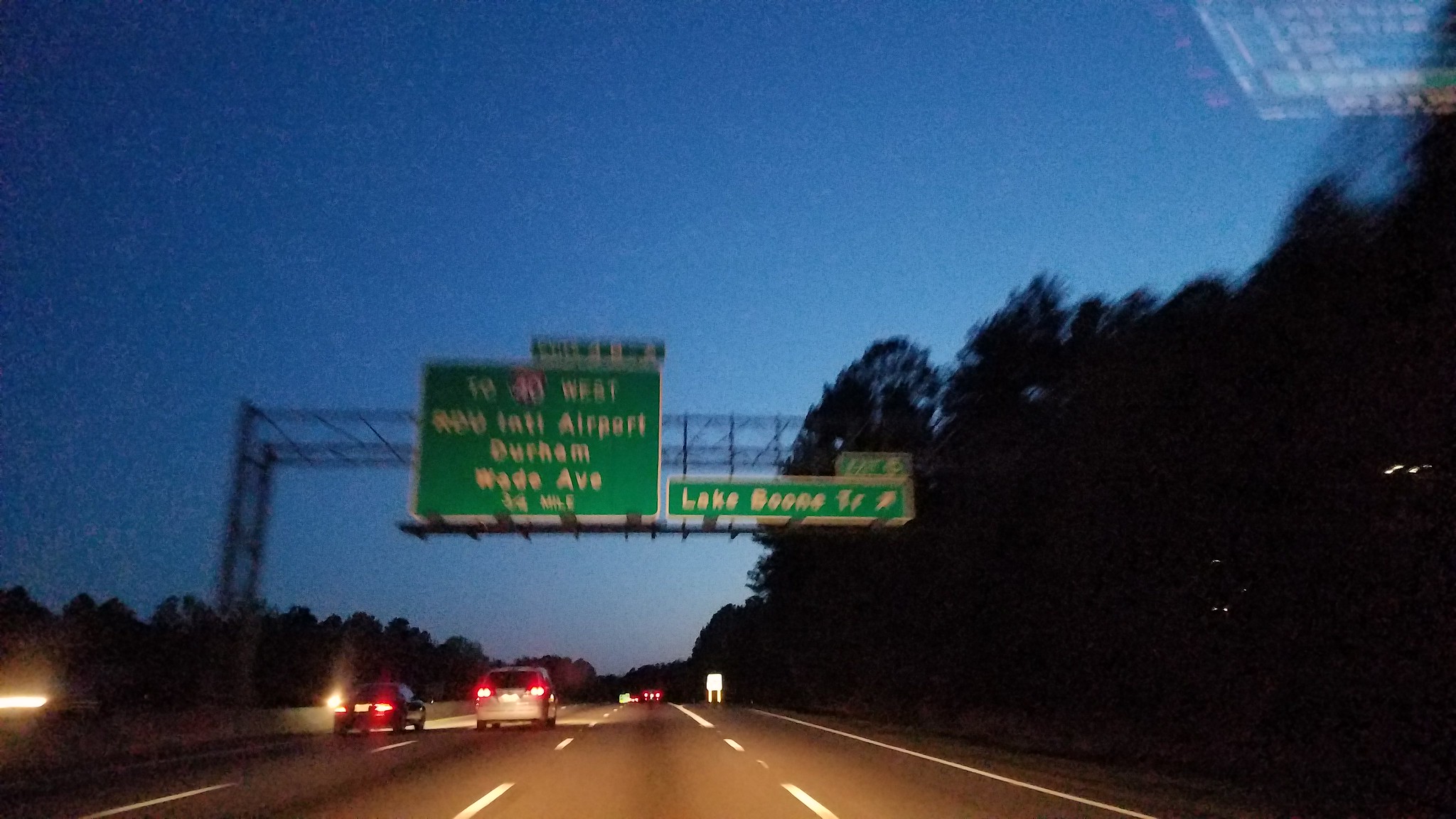Captured during the night, this image presents a view from inside a car traveling on a four-lane highway, as seen through the windshield. The road is outlined by white dashed lines separating each lane. Ahead, two cars with their headlights on can be seen in the left two lanes. Dominating the scene is a pair of green highway signs mounted on a metal scaffold. The larger sign on the left displays "240 West" in bold white letters, followed by directions to "RDU International Airport," and then informs drivers of destinations including "Durham" and "Wade Avenue," which is marked as being "3/4 mile" away. Further to the right, an exit sign marked "Exit 5" indicates the way to "Lake Boone Trail" with a white arrow pointing to the right. The overall ambiance conveys the quiet yet composed nature of night driving, with clear guidance signs leading the way.